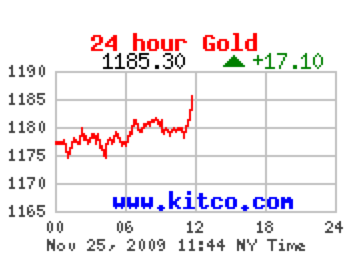The image depicts a chart with a white background, prominently labeled "24 Hour Gold" in red at the top, indicating a tracking of gold prices over a full day. Below this header, the current price is marked as "1185.30" in black font, alongside a green arrow showing a change of "+17.10."

The chart features both vertical and horizontal axes. The vertical axis on the left side ranges from 1165 to 1190, increasing in increments of five. The horizontal axis at the bottom is labeled with time intervals of 0, 6, 12, 18, and 24 hours. Additionally, the bottom of the chart reads "November 25th, 2009, 11:44 NY Time," indicating the date and timestamp of the data.

A gold price trend line, depicted in orange, fluctuates slightly around the 1175 to 1180 range. It eventually peaks at 1185 near the 12-hour mark. The website "www.kitco.com" is displayed in royal blue font at the lower part of the chart, confirming the source of the data.